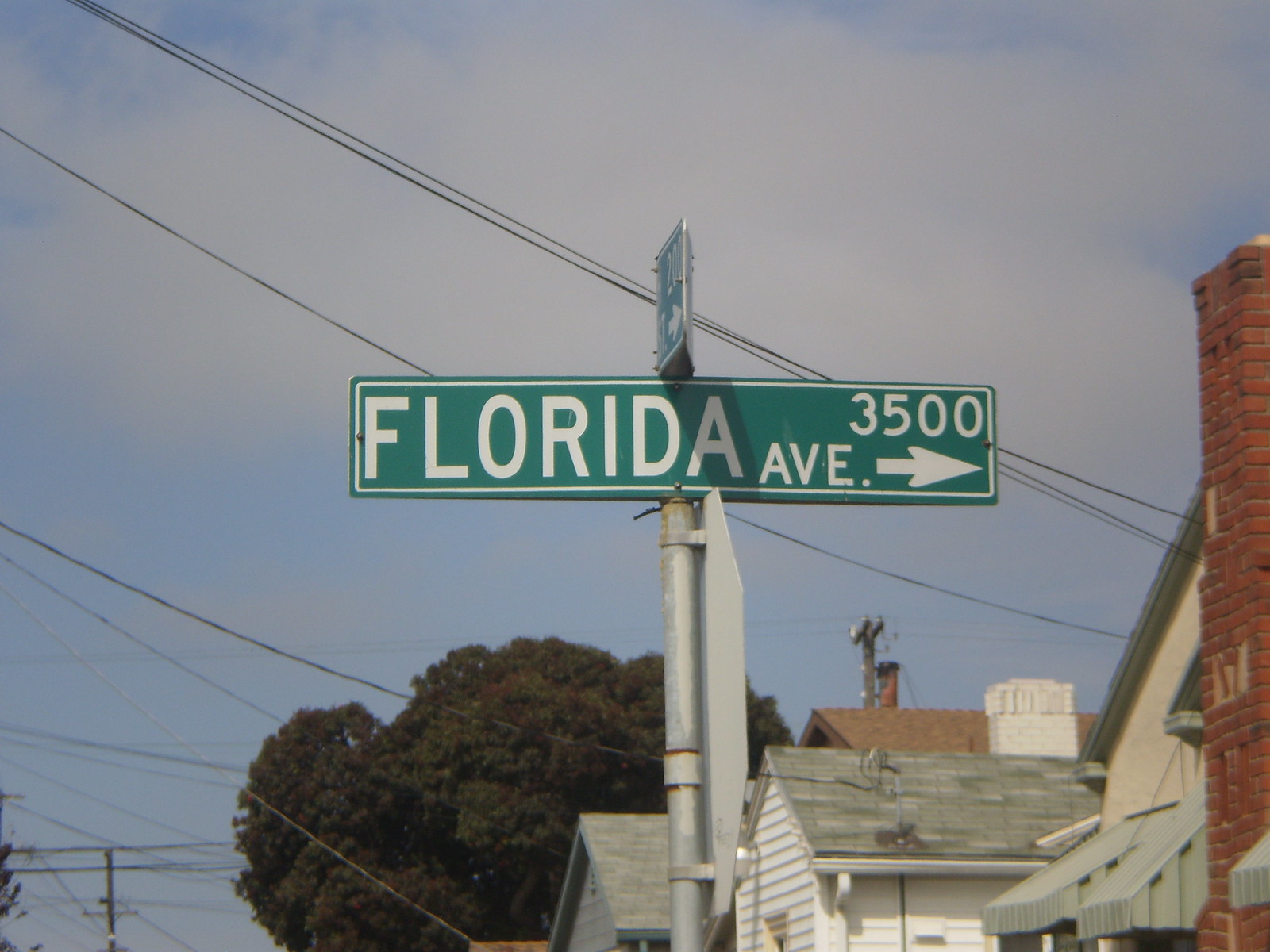The photograph captures a street sign in a residential area, showcasing a green street sign labeled "Florida Avenue," with the number "3500" above it and a white arrow pointing to the right. The sign is mounted above an obscured stop sign seen from the side. The background reveals a partly cloudy sky allowing some blue to peek through. The scene includes multiple utility poles and power lines crisscrossing the view. To the right, several houses with predominantly gray roofs are visible, one of which features a prominent red brick chimney extending down to the ground, although a few bricks seem to be missing. A large tree can also be spotted amidst the houses.